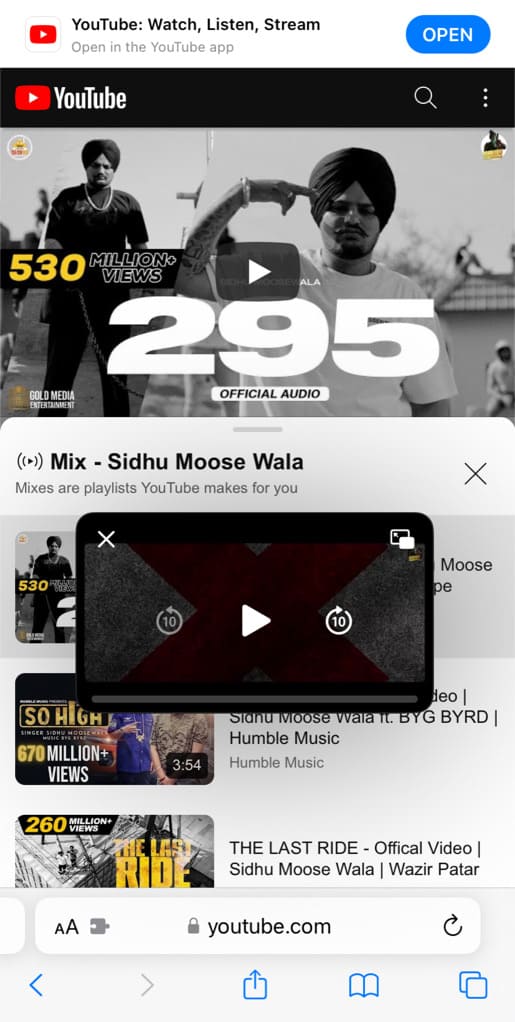This is a screenshot of a YouTube page viewed through a browser on a cell phone, indicated by the banner at the top suggesting to open the app with the message, "Open in the YouTube app: Watch, Listen, Stream." The screen features a pop-up video player with options to minimize, as well as buttons for 10-second rewind, play, and 10-second fast-forward. In the background, a music video titled "Mix Seed Who Moose Wallah" is visible, displaying a person of South Asian origin wearing a head wrap and mimicking holding a gun to their head with their fingers. The video has accumulated 530 million views and is labeled as "295 Official Audio."